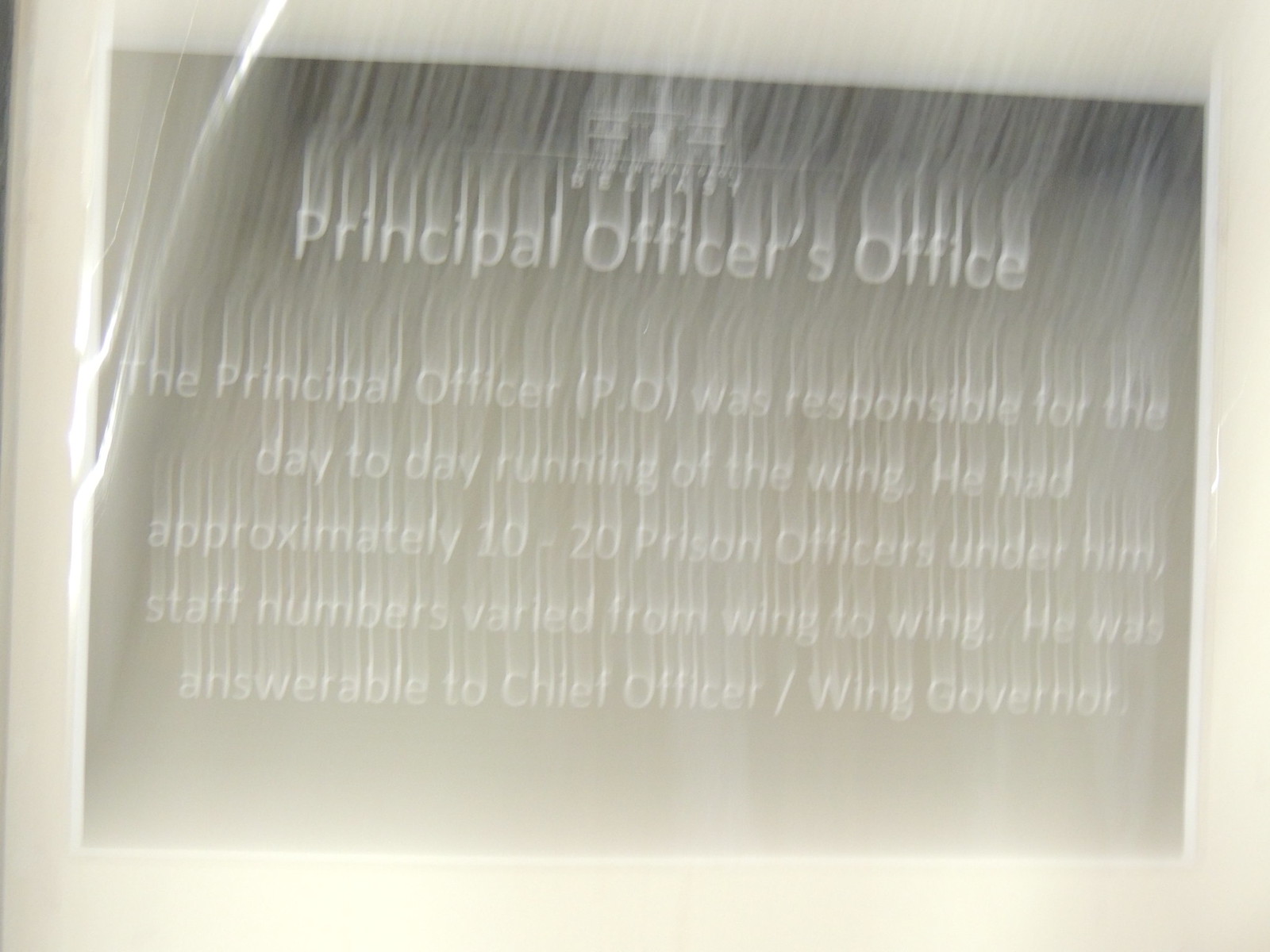This is a photograph of an extremely blurry informational plaque that reads "Principal Officer's Office." The Principal Officer (PO) was responsible for the day-to-day running of the wing and oversaw approximately 10 to 20 prison officers, although staff numbers varied from wing to wing. The PO reported to the Chief Officer/Wing Governor. The sign appears to be made of metal with raised metal lettering and is likely affixed to a stone wall, possibly in a prison or a historical site. The colors visible in the image are various shades of white, beige, and gray. The photo seems to have been taken almost head-on, though it is so distorted and blurry that finer details and the exact environment—whether indoors or outdoors, or the time of day—cannot be determined.